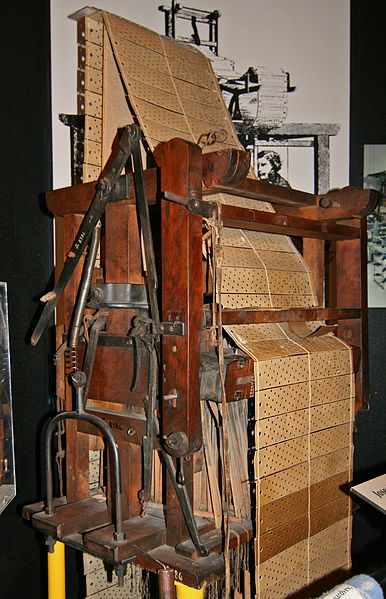The photograph depicts an antique mechanical device, primarily made of thick, solid wooden beams with metal components in the pressing sections. The machine resembles an old printing press but is designed for a different purpose. Instead of paper, it processes long slats of wood, possibly bamboo, organized into rows and tied together with three strings running along the edges and center. These slats, tan in color and patterned into two vertical columns separated by a white line, might be intended for home-use items such as fencing, paneling, or mats. The scene appears to be part of a museum exhibition displaying the machine's function. In the background, there is a black-and-white illustration of the machine, contributing to the historical context. The setup is indoor, highlighting its vintage aspect and educational purpose.